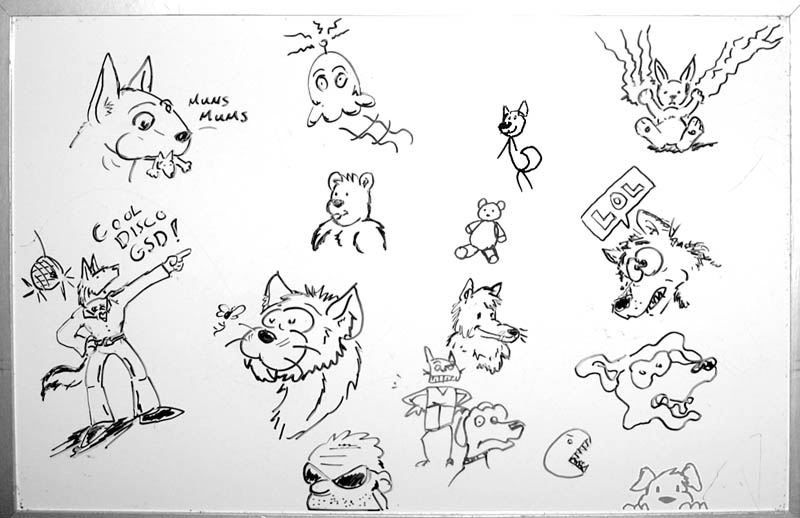This horizontally oriented marker board, framed with silver edges, showcases a myriad of detailed black-and-white cartoon sketches, covering much of its white surface. Dominating the top right is a striking image of a forward-facing bunny, with lightning or energy beams shooting from its paws. Below this electric bunny, a comically clueless-looking dog or wolf utters "LOL" in a speech bubble. Scattered throughout the board are various canine drawings, including a notable scene in the bottom left of a dog or wolf in flared pants and a long-sleeved shirt, pointing right with the phrase "cool disco GSD" beside a hovering disco ball. Toward the middle, a charmingly simplistic teddy bear sketch, reminiscent of childlike drawings, adds to the whimsical array. Among the characters are also fantastical beings like an amoeba-like creature with an antenna emitting some form of energy, an ant-like figure, and another rabbit-like creature with one paw ablaze and the other radiating energy. Overall, this collection of doodles, rendered in pencil or ink, blends imagination and playfulness, with numerous cartoon beasts and sporadic human figures interspersed, creating a dynamic and engaging visual narrative.